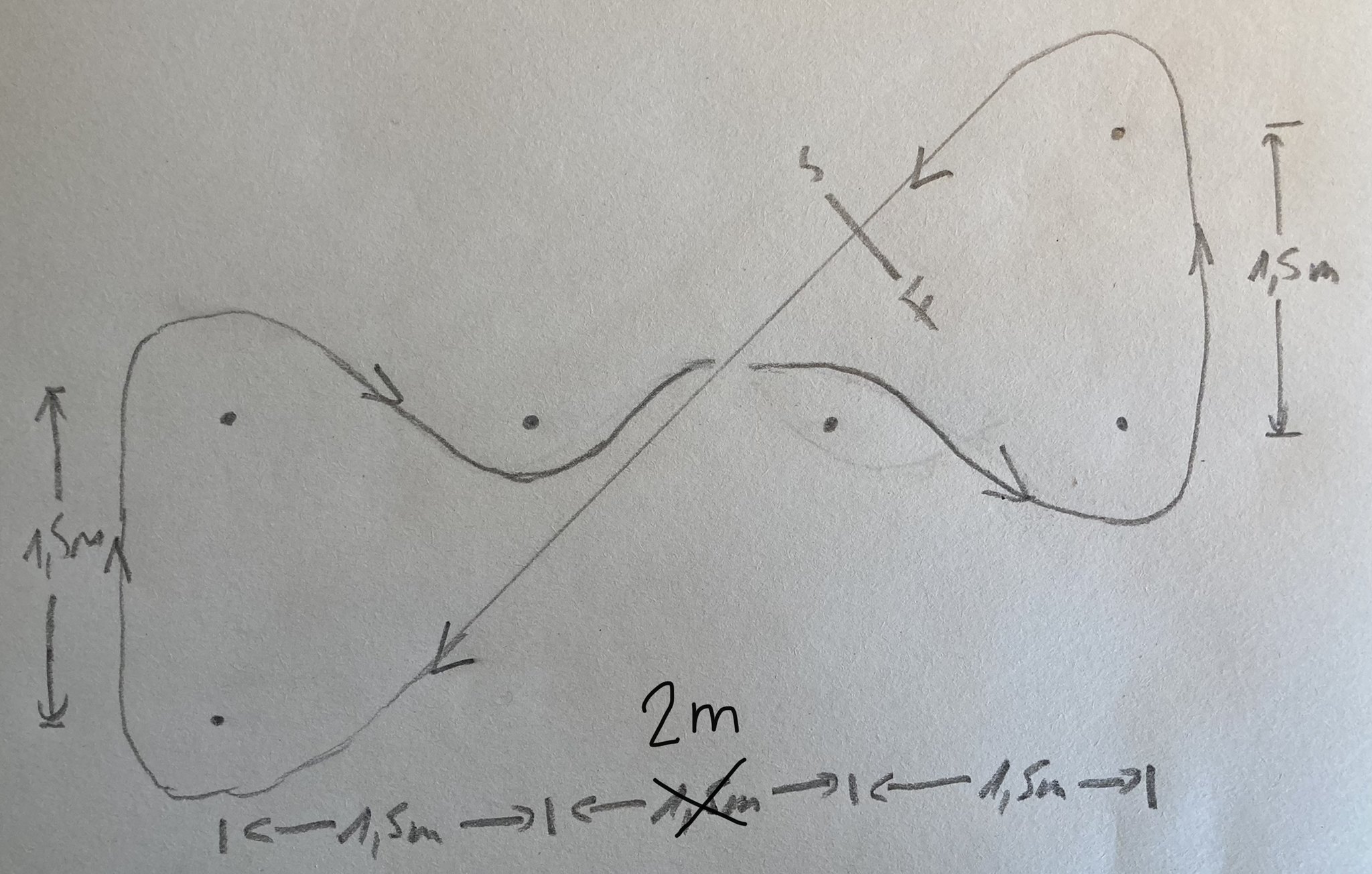The photograph features a piece of white paper oriented sideways, showcasing a combination of pencil and pen markings. The predominant pencil drawing displays a modified figure-eight shape. This figure-eight is distinct because, instead of being entirely smooth, it incorporates a diagonal straight line intersecting part of its curves. The curvy sections are detailed with arrows indicating directionality around the shape.

A short intersecting line within the figure-eight is marked with an "S" at the top and an "F" at the bottom. Various dots are scattered both inside and outside the figure-eight; their significance remains unclear. Notably, on the upper-right side of the figure-eight, there is a notation that appears to read either "S" or "5", followed by "M" (potentially indicating meters). Adjacent to this notation, there is an upward-pointing arrow, a downward-pointing arrow, and a short horizontal line, suggesting this area might represent some kind of scale, possibly denoting "1.5 meters," although it is somewhat illegible.

On the left side of the paper, towards the bottom, there is another scale-like series of markings. This includes a short vertical line on both the left and right, encapsulating a leftward-pointing arrow. Within this area, there is another notation that resembles "A, S, M" or "5M" with additional arrows and short vertical lines. The central part of this sequence indicates a change from "A, 5M" (crossed out) to "2M," again likely suggesting meters. More arrows and short vertical lines follow, ending with another cryptic notation that looks like either "A" or an upside-down "V," combined with "SM."

Overall, the image presents a mix of geometric shapes, directional arrows, and potentially measurement-related notations, forming a cryptic layout that hints at scientific or mathematical content.